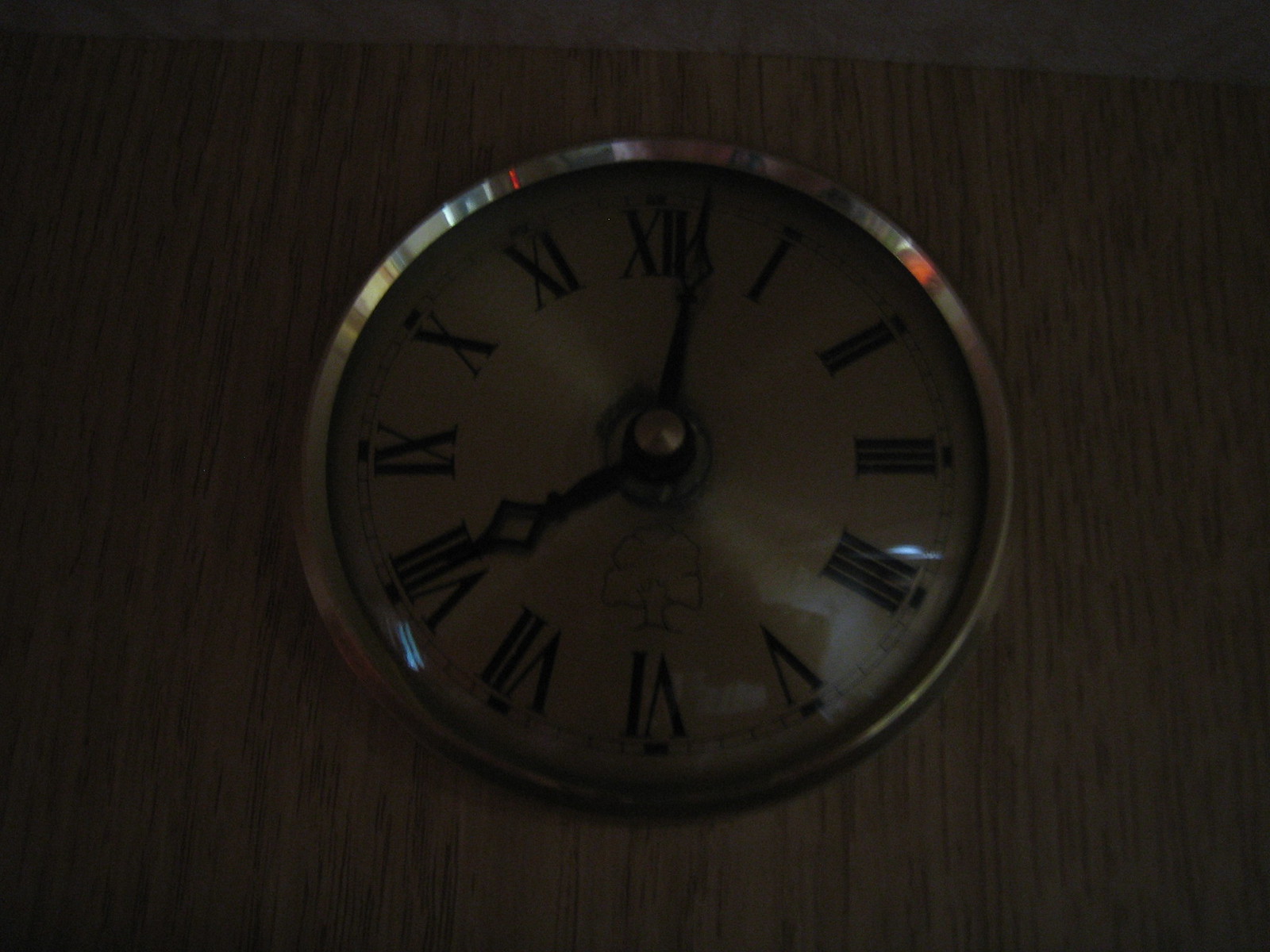This close-up image reveals a meticulously crafted wall clock suspended against a wooden backdrop. The wall's grain runs vertically from the bottom to the top of the image. At the frame's top edge, the muted outline of a roof is faintly visible, though its color remains indiscernible. Central to the composition is a circular clock, prominently featuring a polished chrome-gold rim and base that glisten with a shiny, reflective quality.

The clock face is marked by Roman numerals, tilted in a clockwise direction, adding a dynamic feel to the classic design. Notably, the numeral VI is uniquely upside down in comparison to the upright XII at the top. The hour and minute hands are elegantly designed; both feature pointed diamond shapes at their tips, but the hour hand is distinguished by a larger and thicker diamond, while the minute hand has a smaller, thinner one. The time displayed is precisely 8:02.

Adding a touch of charm, a small tree graphic is situated just below the central bolt that fastens the hands, right above the Roman numeral VI. The meticulous detailing of the clock against the rustic wooden wall creates a harmonious blend of craftsmanship and natural texture.